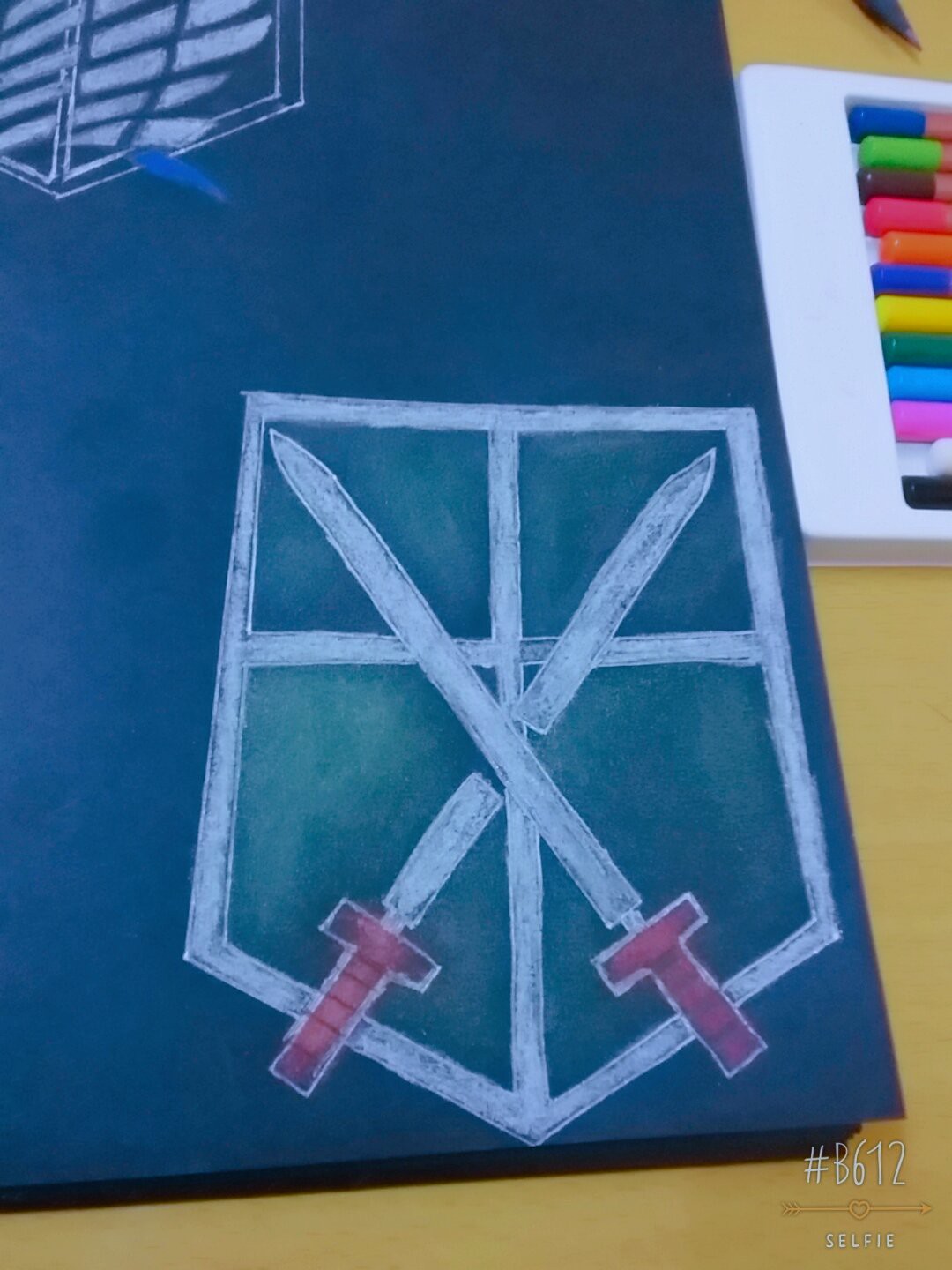A detailed chalk drawing is depicted on a chalkboard that is laid flat on a wooden table. The artwork features a prominent blue shield positioned in the corner of the board. The artist has skillfully shaded the shield to distinguish it from the background, giving it depth and dimension. The shield is designed with a pointed bottom and a flat top. Overlaying the shield, two swords are drawn in a crisscross pattern. One of the swords appears to be severed into two pieces, while the other remains intact. The handles of the swords are vibrant and detailed; the left handle is adorned with pink lines, and the right handle features blue or purple lines. 

In addition to the main drawing, the table holds several markers, indicating the tools used for this artwork. Above the blue shield, there is another partially completed shield drawn in white chalk with a notable blue mark on it. The entire scene captures the artist's process and the evolving nature of their work.